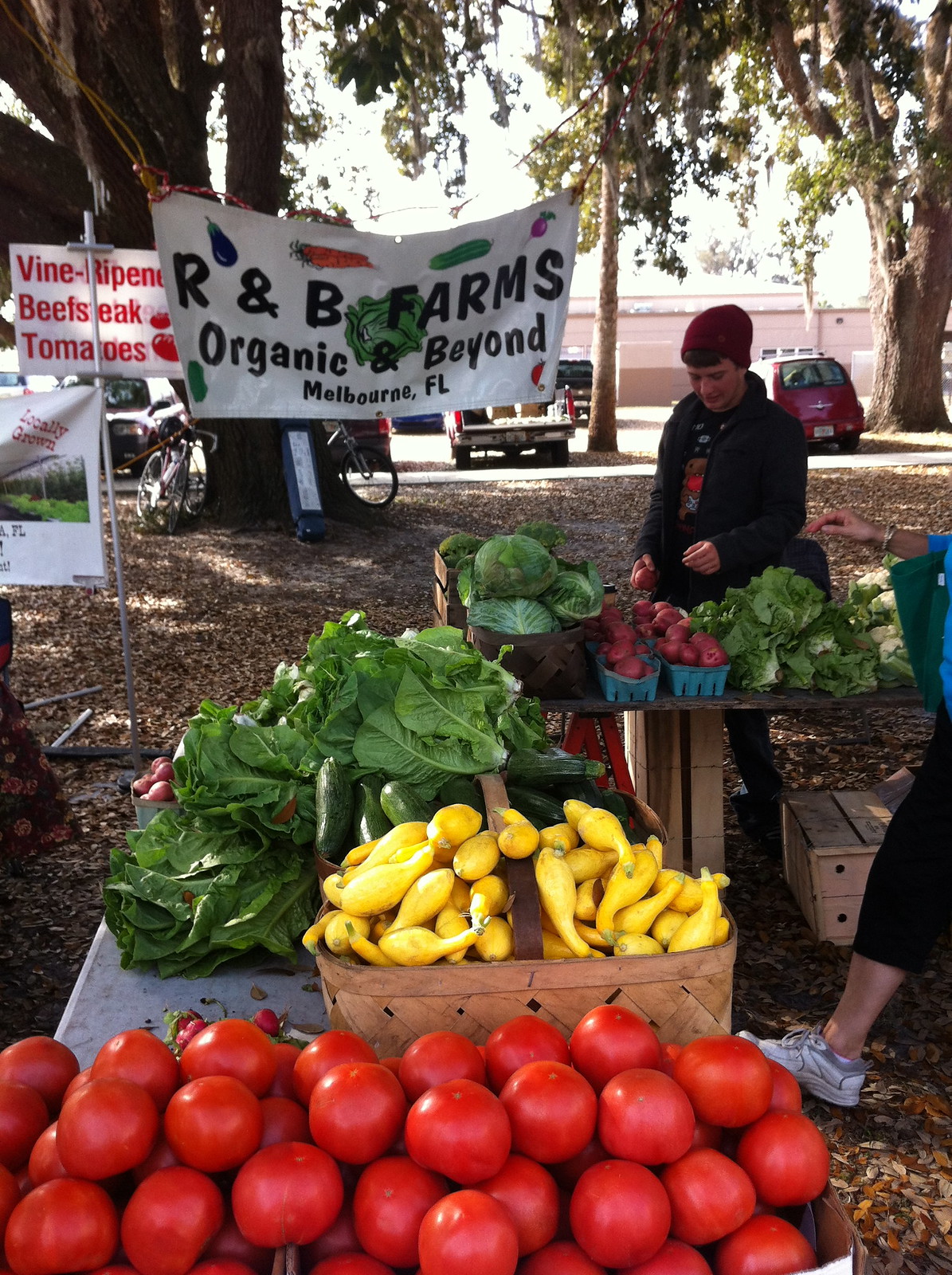The image portrays an outdoor organic vegetable stand, likely part of a farmer's market, set up amidst a ground covered in a carpet of yellow and brown leaves. Centered in the setup is a multi-tier display that starts with a large box filled with very large red tomatoes at the bottom. Above it, a wicker basket holds yellow squashes, while green leafy vegetables occupy a higher level. To the right, a wooden table supports blue containers brimming with red apples, flanked by more green leafy vegetables on both sides.

In the background, a banner hangs from the trees, featuring a white backdrop with blue letters that read "RNB Farms, Organic and Beyond, Melbourne, Florida." Adjacent to the banner is a white square sign with red letters that lists "Vine, Spend, Beet, Steak, Tomatoes." 

A woman, characterized by her downturned head, wears a dark orange beanie and a black coat, standing behind the vegetables with both hands in front of her. To the right, partially visible, is another person whose leg, clad in black pants and a white shoe, extends towards the squash. The market atmosphere is reinforced by the presence of another man wearing a maroon beanie, black coat, and black shirt featuring a game character, likely "Super Meat Boy." He is perusing the vegetable stand, suggesting a communal experience in this picturesque setting studded with nature’s bounty.